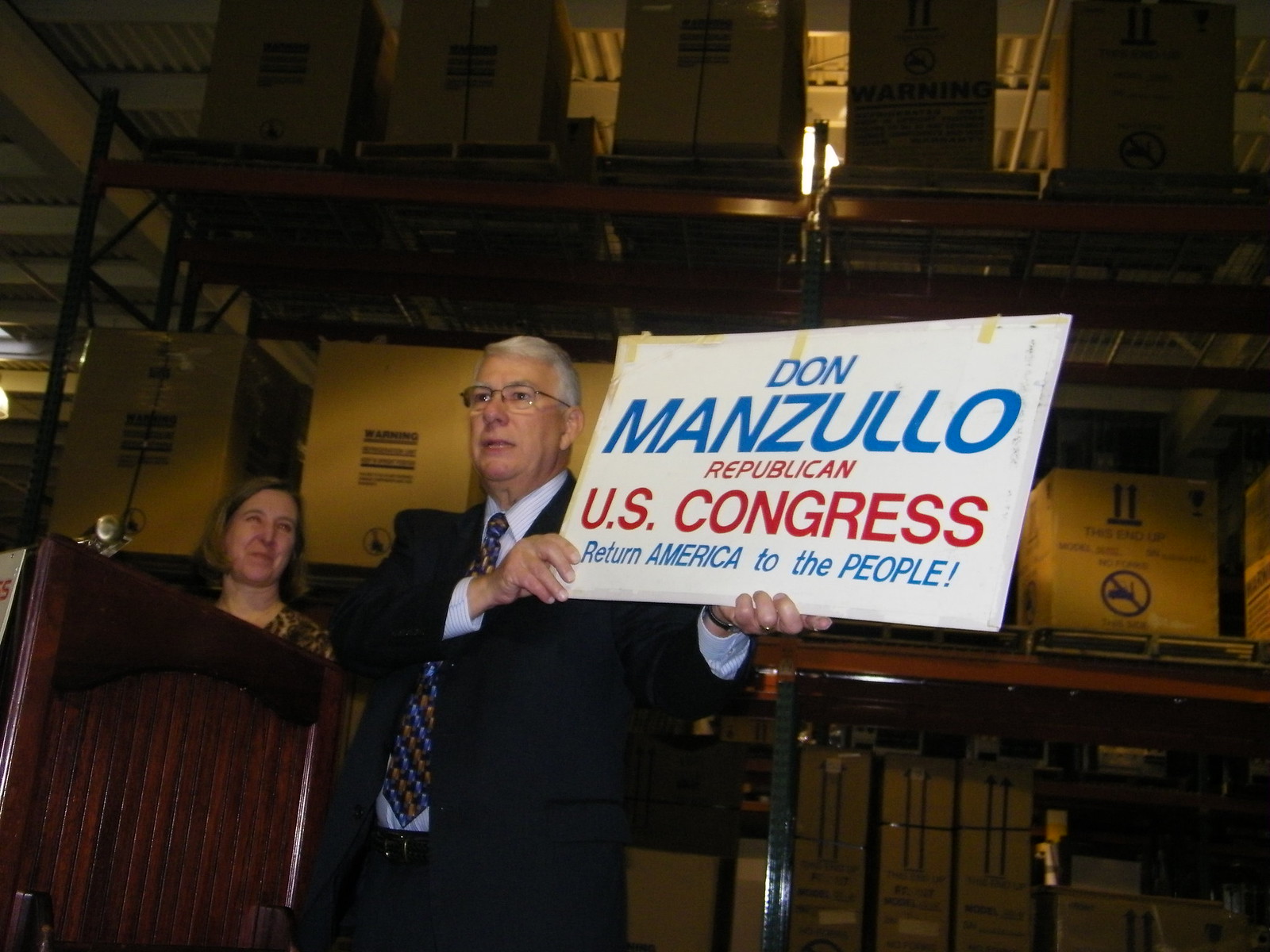The large square image depicts Don Manzullo, a politician, dressed in a black suit and a colorful blue and orange patterned tie, standing at the center. He holds a horizontally-aligned, worn white sign with black, red, and blue lettering that reads, "Don Manzullo, Republican U.S. Congress, Return America to the People." Manzullo, characterized by his short gray hair and small wire-rimmed glasses, gazes off towards the left. The setting appears to be a gold-walled room, possibly an auditorium or factory, evidenced by the presence of machinery and boxes in the background. A dark brown podium is visible in the lower left corner with a woman standing behind it. She has short brown hair and wears a black and gold top, staring intently at Manzullo, further emphasizing the campaign atmosphere of the scene.